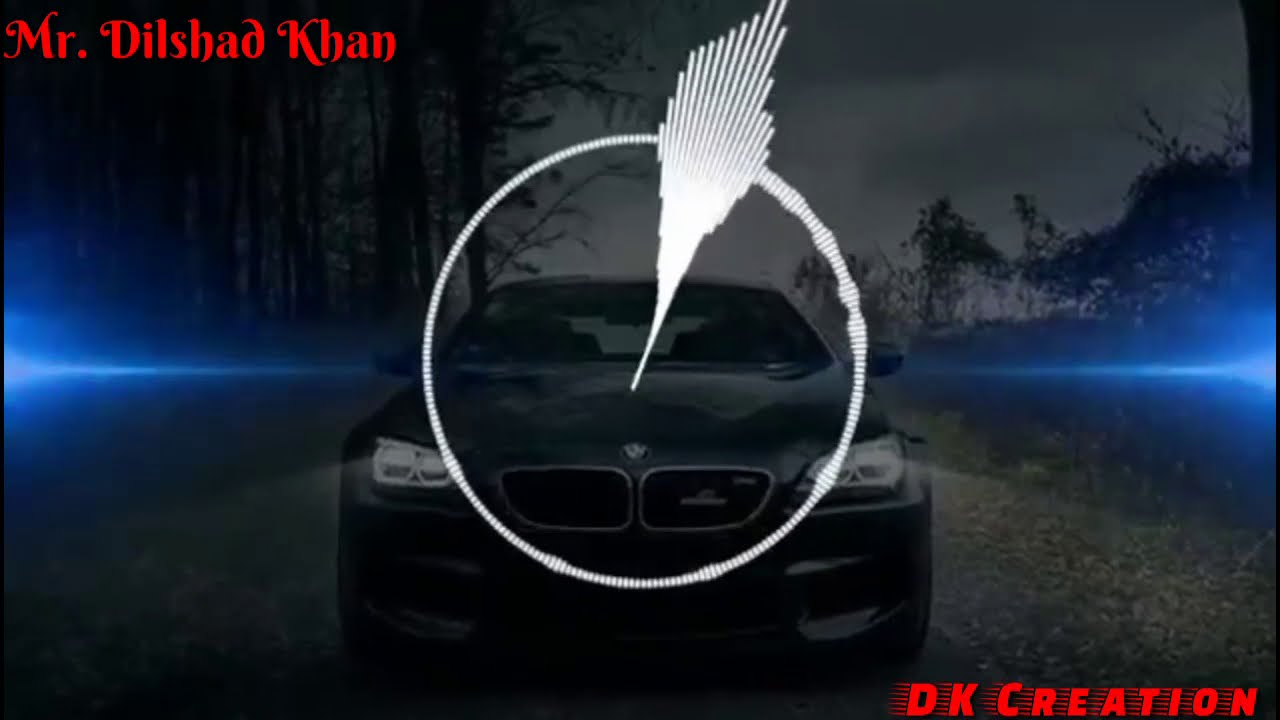The image appears to be a dark, stylized graphic likely used as a YouTube video thumbnail. Dominating the background is a BMW car, barely visible through the dark shades of gray. The scene is set on a dirt or leafy road surrounded by a forest with dense trees on both the left and right. The overcast sky above is mostly gray and cloud-filled, hinting at impending rain. Blue streaks of light radiate from the left and right edges of the image, adding a surreal touch. Positioned in the center is a graphic symbol: a circular design with an intricate digital feather-like illustration emanating from it. In bold red fantasy font, the text "Mr. Dilshad Khan" is prominently displayed in the top left corner, while the bottom right corner features "DK Creation" in an action-style red font. Overall, the image is moody and stylized, with elements carefully balanced to create a coherent and visually striking composition.